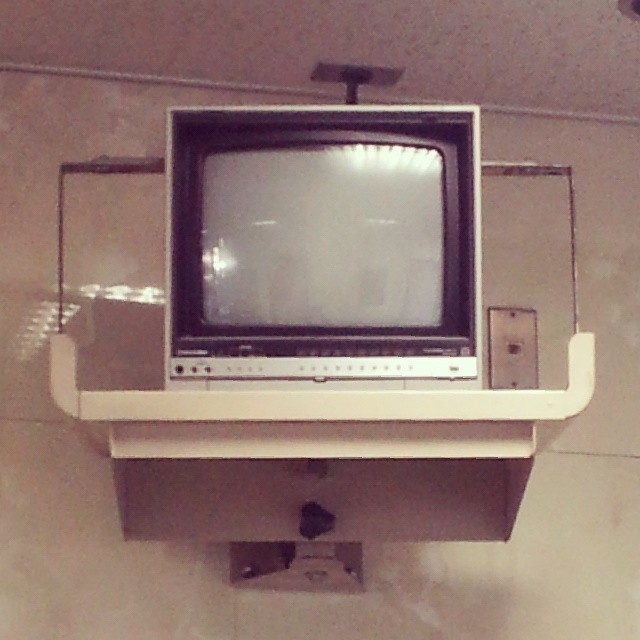This detailed photo captures an aged television set, reminiscent of the early models from decades past. Positioned centrally in a wide vertical rectangular shot, the TV rests on a unique white plastic shelf that appears to be mounted both to the wall and the ceiling with a metal attachment. The shelf, which curves upward at the sides, includes a hollow rectangular section beneath it for added support. The monitor itself is square and predominantly silver, framed in black plastic around the screen. The screen is a muted gray, reflecting the overall faded color palette of the image which gives a black-and-white impression. Below the screen, the TV features a wider silver strip with an array of buttons, and further down, another black strip likely containing identifying information about the TV. The rigid shelf structure is augmented with a silver hook that curves around the TV and extends from the wall mount to the ceiling, ensuring the TV is securely suspended. The background wall, instead of a bright white, displays a dull tan or light brown hue, enhancing the vintage feel of the scene. An additional detail is a visible switch to the lower right of the TV in the background.